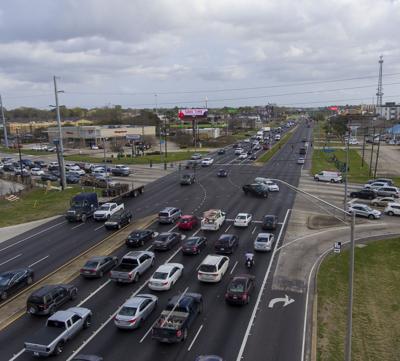The image shows an overhead view of a busy highway intersection set in a residential area. The highway features multiple lanes—a larger five-lane section on one side and a narrower two-lane section on the other. There are both left-turn lanes and straight-through lanes, indicating a complex traffic pattern. Numerous cars of various types are navigating in different directions, suggesting peak traffic conditions. Surrounding the highway are several buildings, including what might be auto shops or small shopping centers. The scene lacks visible traffic lights, reinforcing the idea that this is a highway. The sky is open and mostly clear, with no tall buildings around, giving the impression of a more open, semi-rural landscape. The presence of multiple cars at the intersection and along the highway hints at a well-traveled area despite the open surroundings. The possibility of the image being generated by AI is suggested, as some cars appear misaligned or facing the wrong direction.